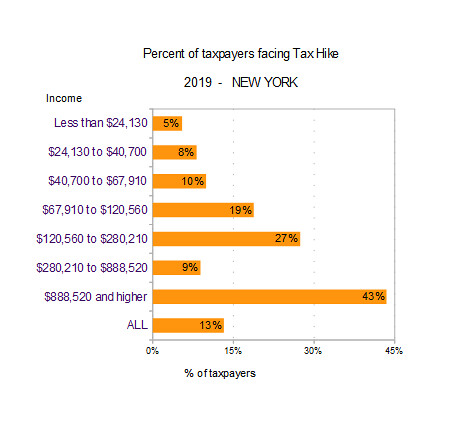This image is a detailed bar graph titled "Percent of Taxpayers Facing Tax Hike, 2019, New York." The background is white, and the bars are orange. The graph categorizes income ranges on the left, with accompanying percentages of taxpayers in each category who are facing a tax hike. 

- Income less than $24,135: 5% 
- Income $24,130 to $40,700: 8% 
- Income $40,700 to $67,910: 10% 
- Income $67,910 to $120,560: 19% 
- Income $120,560 to $280,210: 27% 
- Income $280,210 to $888,520: 9% 
- Income $888,520 and higher: 43% 
- For all taxpayers: 13%

The bar graph features large, clearly defined orange bars extending to the right to represent these percentages, with the percentages listed at the bottom of the graph: 0, 15, 30, and 45%. Additional text at the bottom of the graph reiterates that these percentages represent the "percent of taxpayers."